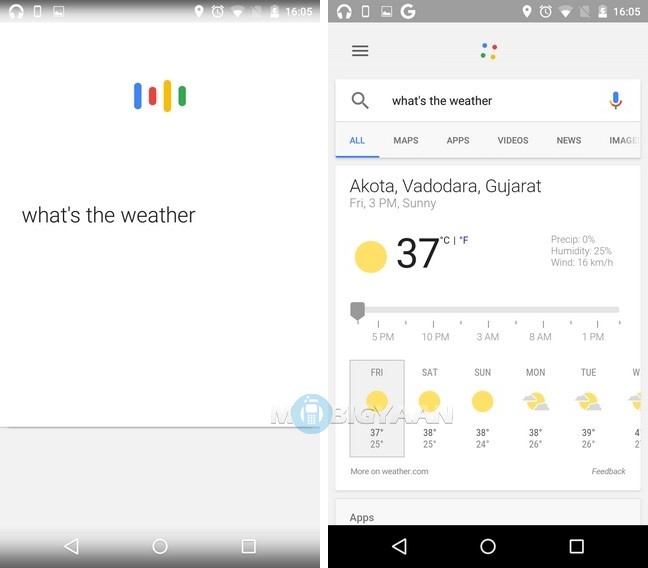The image is divided into two sections, both displaying information on a smartphone and set against a white background. On the left side, there is a conversation with Google Assistant. At the top center of this section, the Google Assistant icon is depicted as four vertical lines in blue, red, yellow, and green, indicating that the assistant is listening. The user has asked, "What's the weather?" 

On the right side of the image, the response is shown, sourced from a Google search page. The search bar at the top reads "What's the weather?" Below the search bar, several tabs are visible—All, Maps, Apps, Videos, News, Images—with the "All" tab highlighted in blue. The weather information is specific to Akota, Vadodara, Gujarat, and details the weather for Friday at 3 p.m., depicting a sunny condition with a temperature of 37 degrees Celsius. To the right, it indicates zero precipitation, 25% humidity, and a wind speed of 16 kilometers per hour. A yellow icon next to the 37 degrees Celsius represents sunny weather.

Further down, there's an hourly weather forecast from 5 p.m. to 1 a.m., viewable via a slider. Below this, a weekly weather forecast is provided. For Friday, the high is 37 degrees and the low is 25 degrees. Saturday's forecast shows a high of 38 degrees and a low of 25 degrees. Sunday sees similar temperatures with a high of 38 degrees and a low of 24 degrees. Monday projects a high of 38 degrees and a low of 26 degrees, while Tuesday expects a high of 39 degrees and a low of 26 degrees.